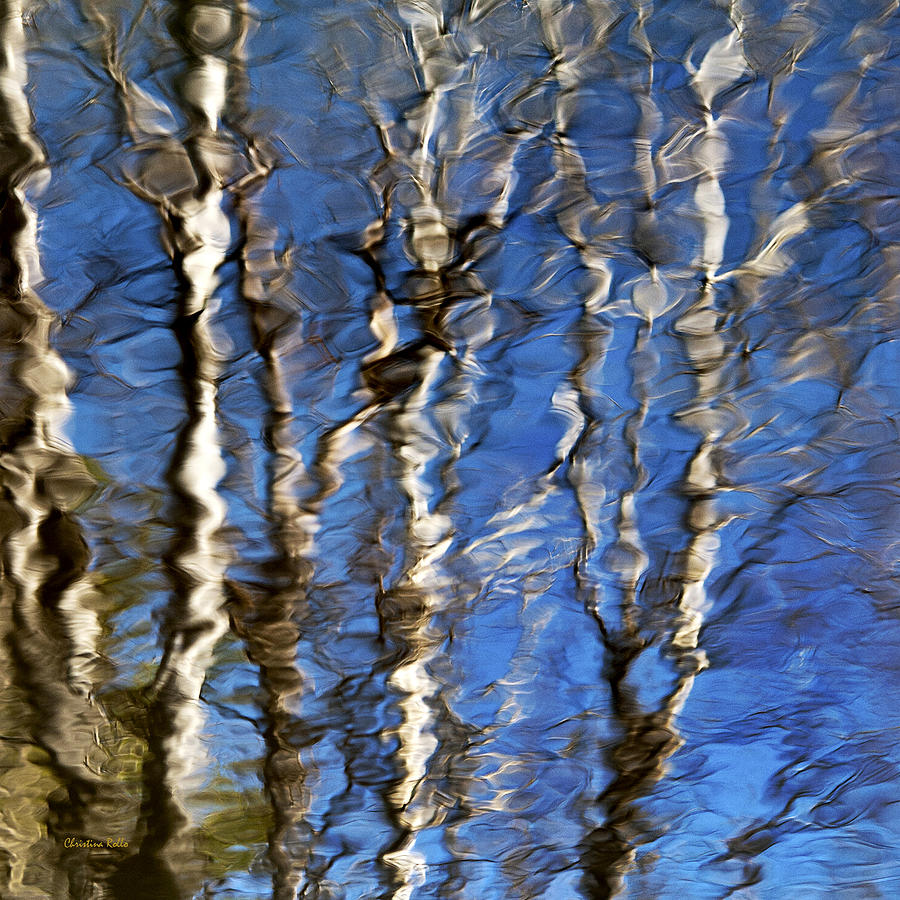The image is a detailed painting that resembles the reflection of birch trees on the surface of a disturbed, rippling body of blue water. Stretching vertically across the entire frame are the distorted, squiggly reflections of white and dark brown tree trunks, likely birch trees, interspersed with some smaller branches. A few green leaves are discernible in the bottom left corner, adding a touch of color amidst the abstract representation. The lower left of the image notably features a watermark with the name "Christina Rollo". The overall impression is one of a serene yet artistically distorted natural scene, highlighted by the bright blue of the water and sky.